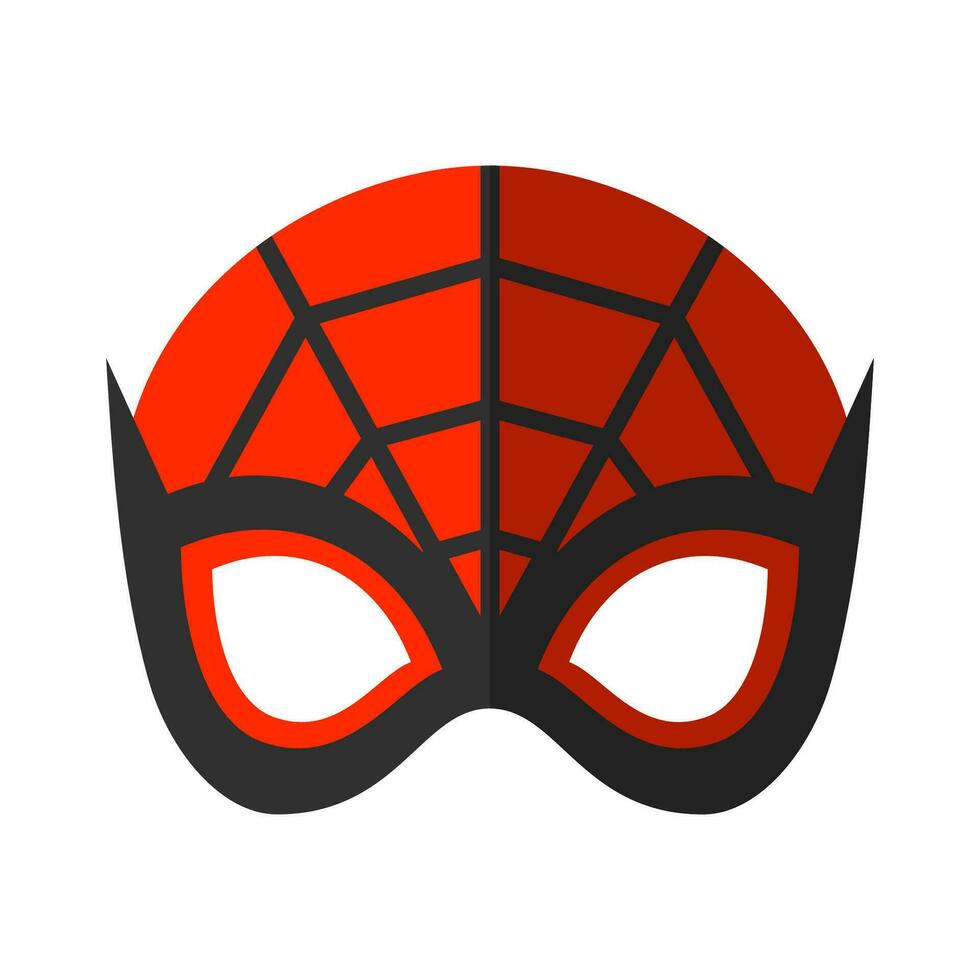This image depicts a minimalistic drawing of Spider-Man's mask set against a completely white background. The mask features a distinctive red and black color scheme. The top of the head is red, adorned with black spider-webbing lines that radiate from the bridge of the nose outward, creating an intricate pattern. Around the eyes, there is a striking black outline which forms into sharp points at the upper corners of each eye, with the inner border colored red. The eyes themselves are stark white, adding a vivid contrast to the mask. The overall design emphasizes the iconic Spider-Man aesthetic with its simplified yet detailed elements.